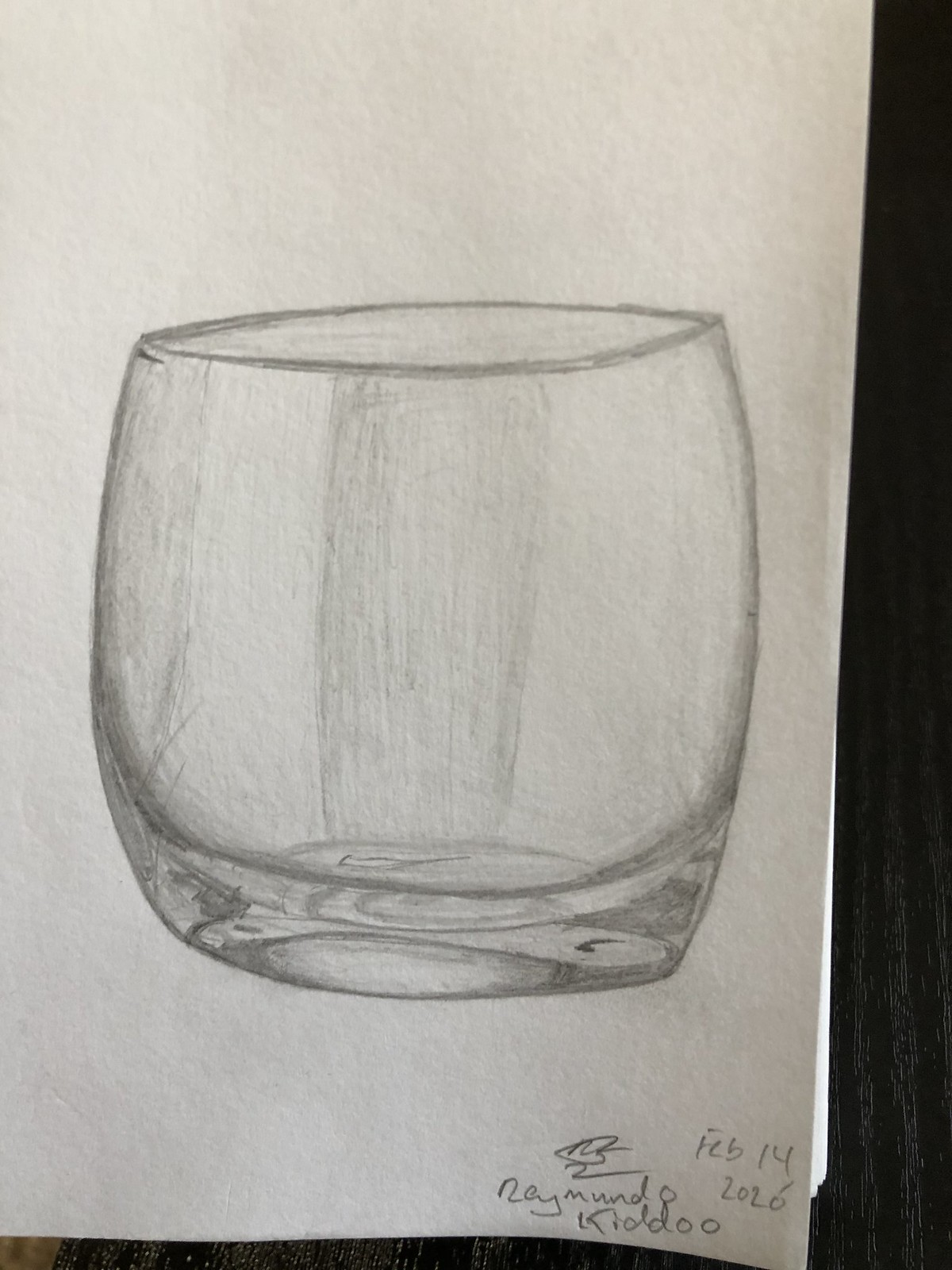This pencil drawing on a white piece of paper depicts an elegantly sketched, small drinking glass that is distinctly made of glass. The glass, rounded at the top and bottom and tapering towards the center, showcases detailed craftsmanship with visible rings around its center base indicative of its blown glass origin. Notably, the glass has slight irregularities - it curves more on the bottom left, while the bottom right is slightly pointy. The drawing, monochromatic and shaded in gray tones, occupies a significant portion of the image, emphasizing its meticulous detail. The artwork is prominently signed by "Naimundo Kudo" at the bottom right corner and dated February 14, 2024. A dark gray strip forms the background, enhancing the sketch's prominence, while the overall piece is set against a backdrop that mimics a black woodgrain table.